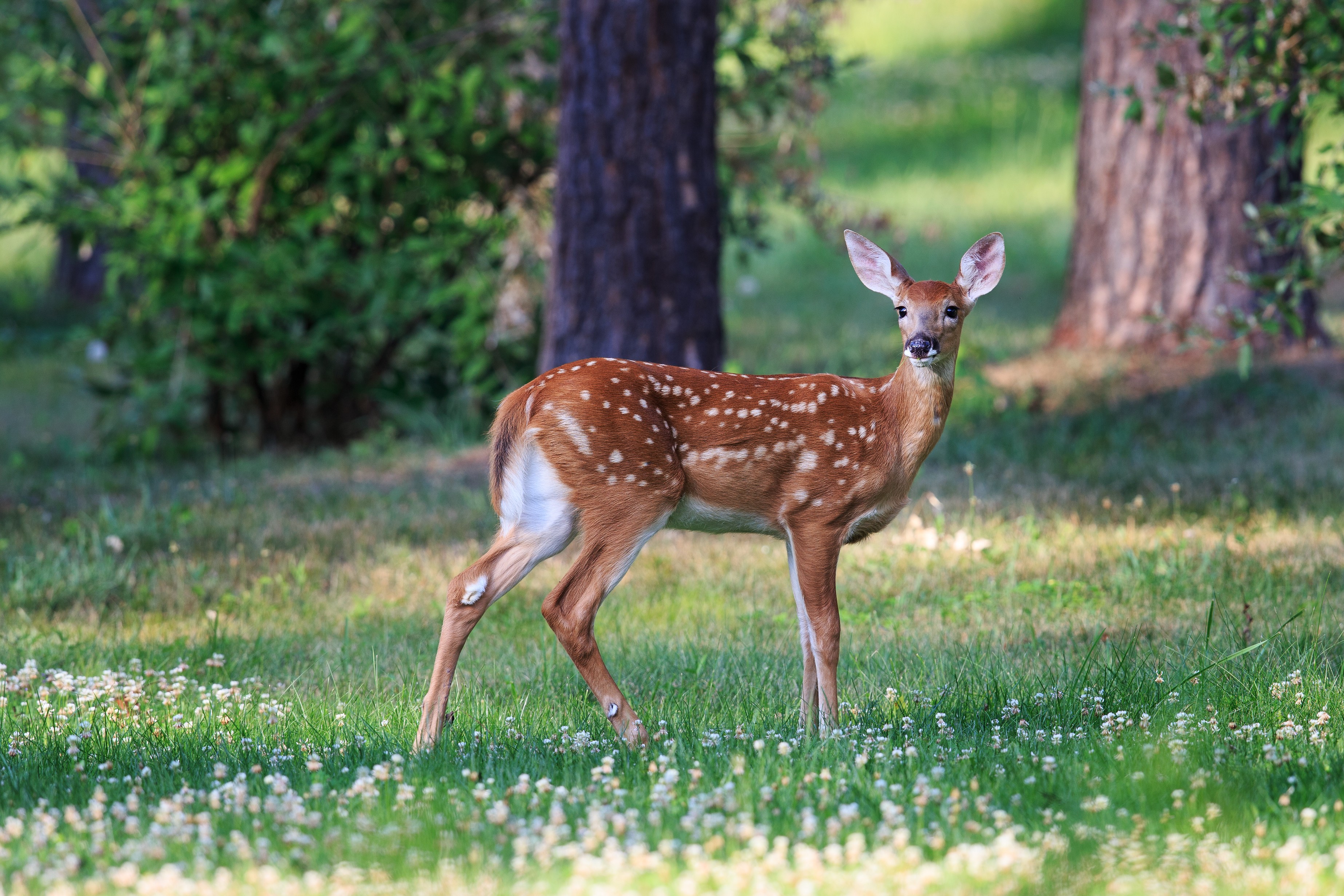This detailed color photograph, oriented horizontally, captures a picturesque scene with a young deer as the central subject. The deer, positioned in the middle of a lush, green field adorned with blooming wildflowers, is standing in profile facing the right. It has golden-brown fur accented with delicate white spots along its sides and back, a white underside, and slender brown legs. The deer’s large, attentive ears are pointed skyward, and it gazes directly at the camera with its black nose prominent.

In the background, the image features two substantial tree trunks, possibly oaks, which are only partially visible, adding a woodsy ambiance to the scene. A sizable green bush is noticeable on the left side of the image, and more grass and wildflowers extend into the distance, enhancing the depth and natural beauty of the setting. The overall style of the photograph leans towards representational realism, vividly capturing the serene, forest-like environment surrounding the peaceful deer.